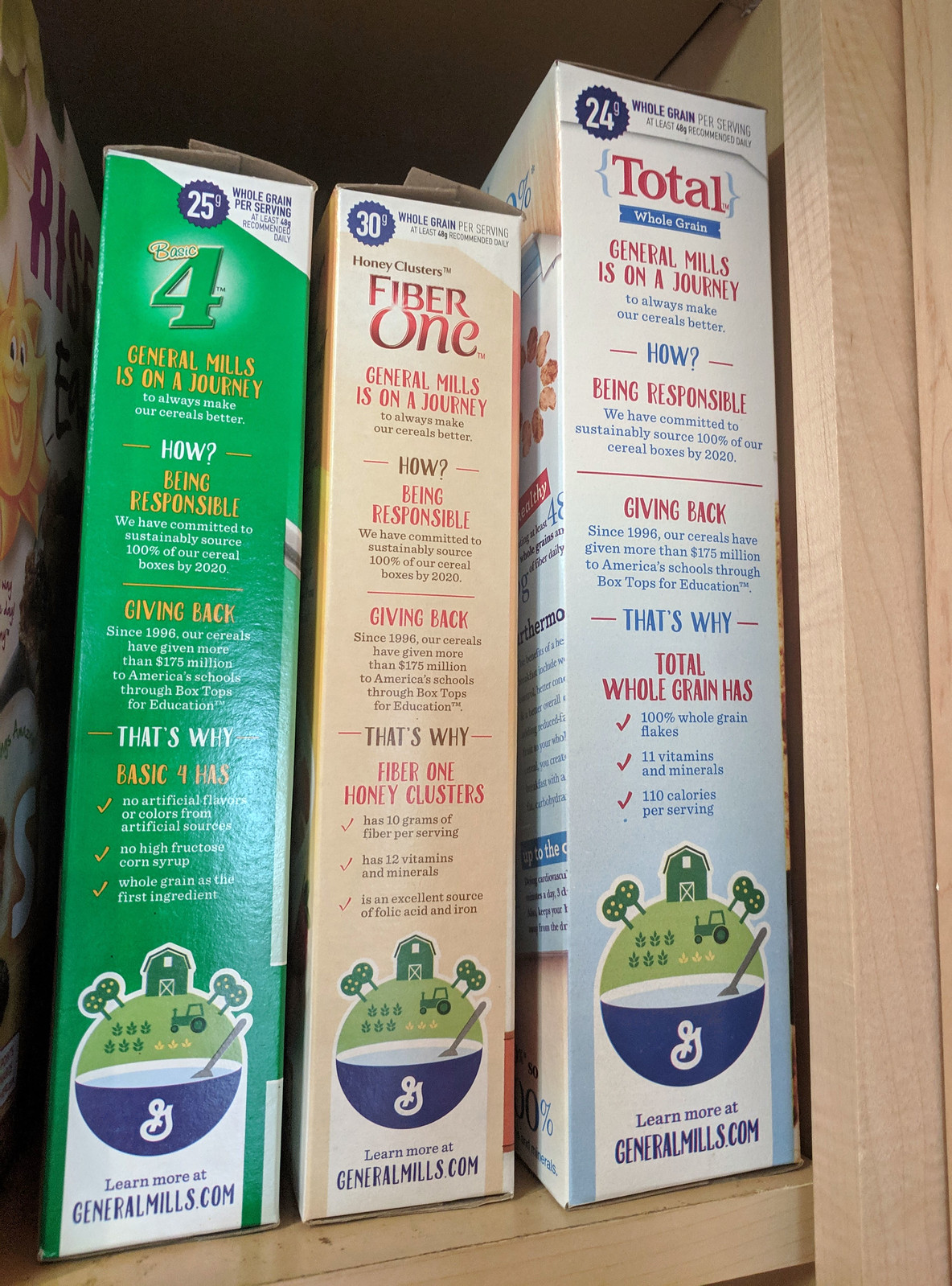This image shows three cereal boxes neatly arranged on an oak-colored wooden shelf inside a cabinet, which is visibly open on the right side. The leftmost box has a green side with the number '4' prominently displayed. This box features details about its health benefits, including the General Mills symbol at the bottom, and depicts a blue cereal bowl marked with a 'G' and a spoon, set against a backdrop of green grass, trees, and a barn. Adjacent to it is a peach-colored Fiber One cereal box, also from General Mills. The third box is a white Total cereal box, taller than the rest, and similarly bears the General Mills logo. Together, these boxes form a tidy row inside the brown wooden cabinet.